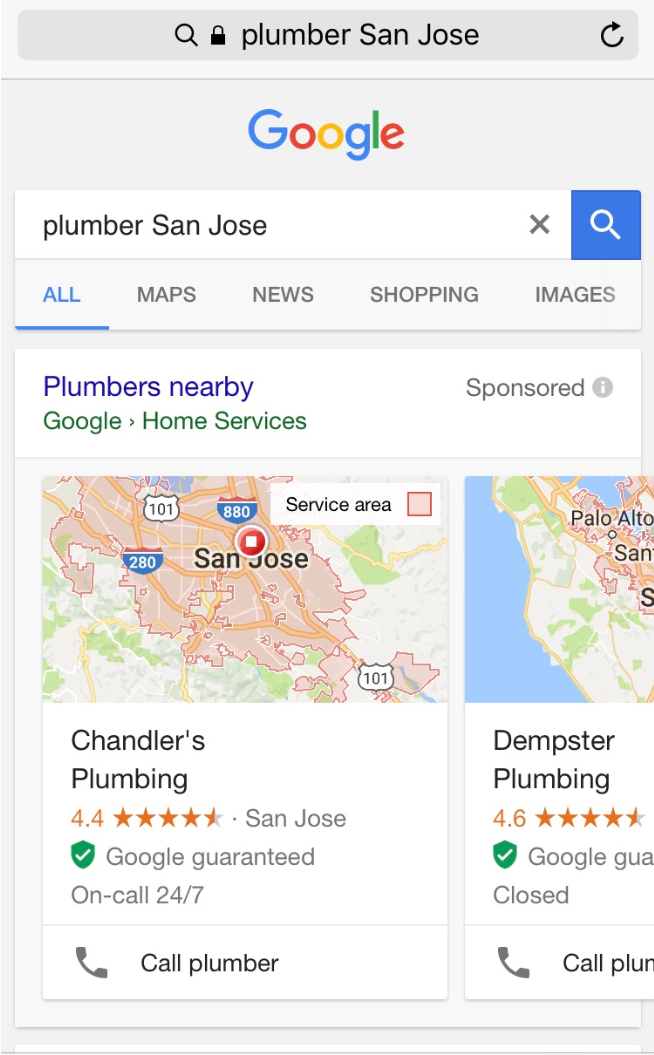The screenshot depicts a website interface, specifically that of a Google search results page. At the top, there is a light gray search bar featuring a black magnifying glass icon. Adjacent to it, there's an icon of a locked keypad. The search input area displays the query “Plumber San Jose,” with both "S" and "J" capitalized.

Below the search bar, there’s a refresh icon followed by the Google logo in its traditional multicolored format. The main search bar is white and again contains the text “Plumber San Jose.” On its right side, there is an "X" for clearing the search and a blue square with a white magnifying glass inside it for executing the search.

Underneath the main search bar, navigation tabs labeled "All," "Maps," "News," "Shopping," and "Images" are visible. The "All" tab is highlighted with blue text and an underline.

A promotional banner reads "Plumbers nearby, Google home services" in green text, accompanied by the term "Sponsored" within a gray circle containing the letter "i."

Two highlighted service panels are shown below. The first panel features Chandler's Plumbing, detailing its service area as San Jose, boasting a 4.4-star rating, marked with the "Google Guarantee," and offering 24/7 availability with a "Call Plumber" button. The second, partially visible panel, lists Dempster Plumbing with a 4.6-star rating, also Google Guaranteed, noted as "Closed," with a "Call Plumber" button.